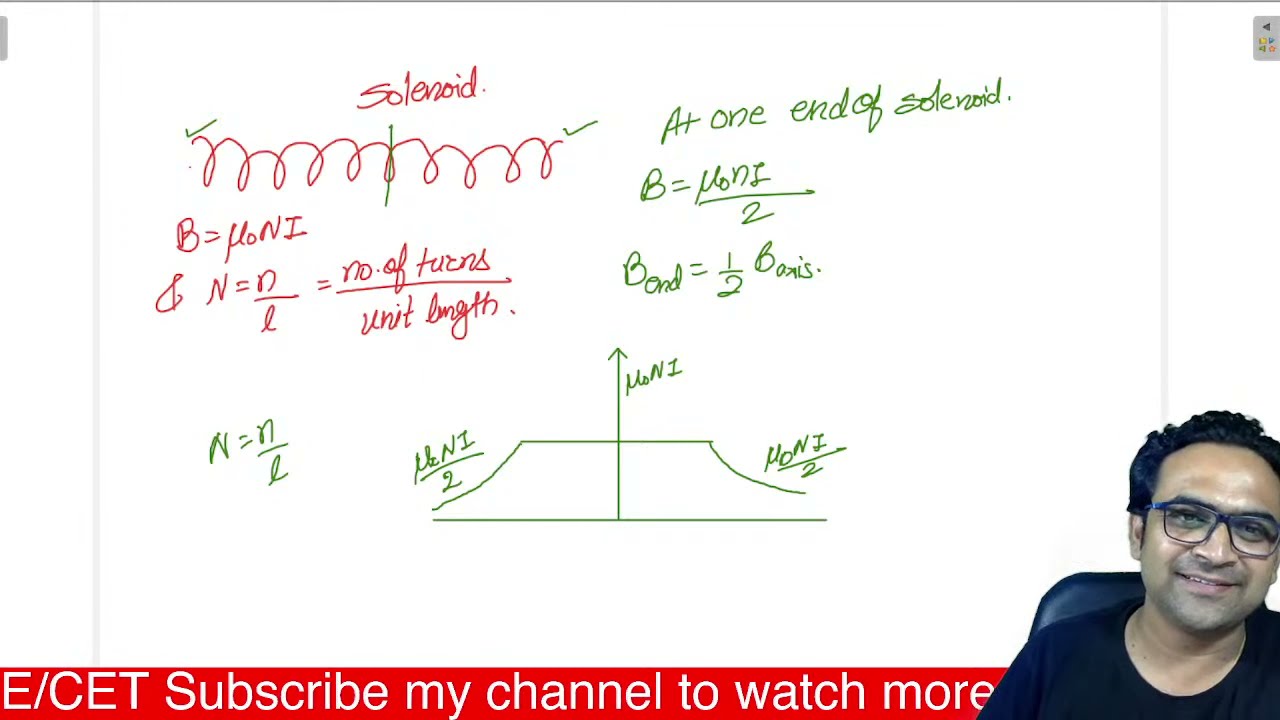The wide rectangular image is a screenshot of an educational video, specifically focused on mathematical equations related to electrical engineering and solenoids. The background is predominantly white, with thin gray strips running from top to bottom on either side. Central to the image are handwritten mathematical equations in various colors - red, green, and purple - such as "A+1" and "B = μ₀ n/2." Additional notes about a solenoid appear, including a drawing of it resembling a spring. In the upper left, it reads "solenoid," while specific equations and definitions, like "n = N/L" and the number of turns per unit length, are visible.

An Indian or Pakistani man appears in the bottom right corner, wearing black-framed glasses and a black T-shirt, seated in a black leather chair. A red banner at the bottom of the image reads "E/CET Subscribe to my channel to watch more," encouraging viewers to stay tuned for future content. The detailed mathematical notations and the presence of the video host suggest this is part of a tutorial on solenoids.